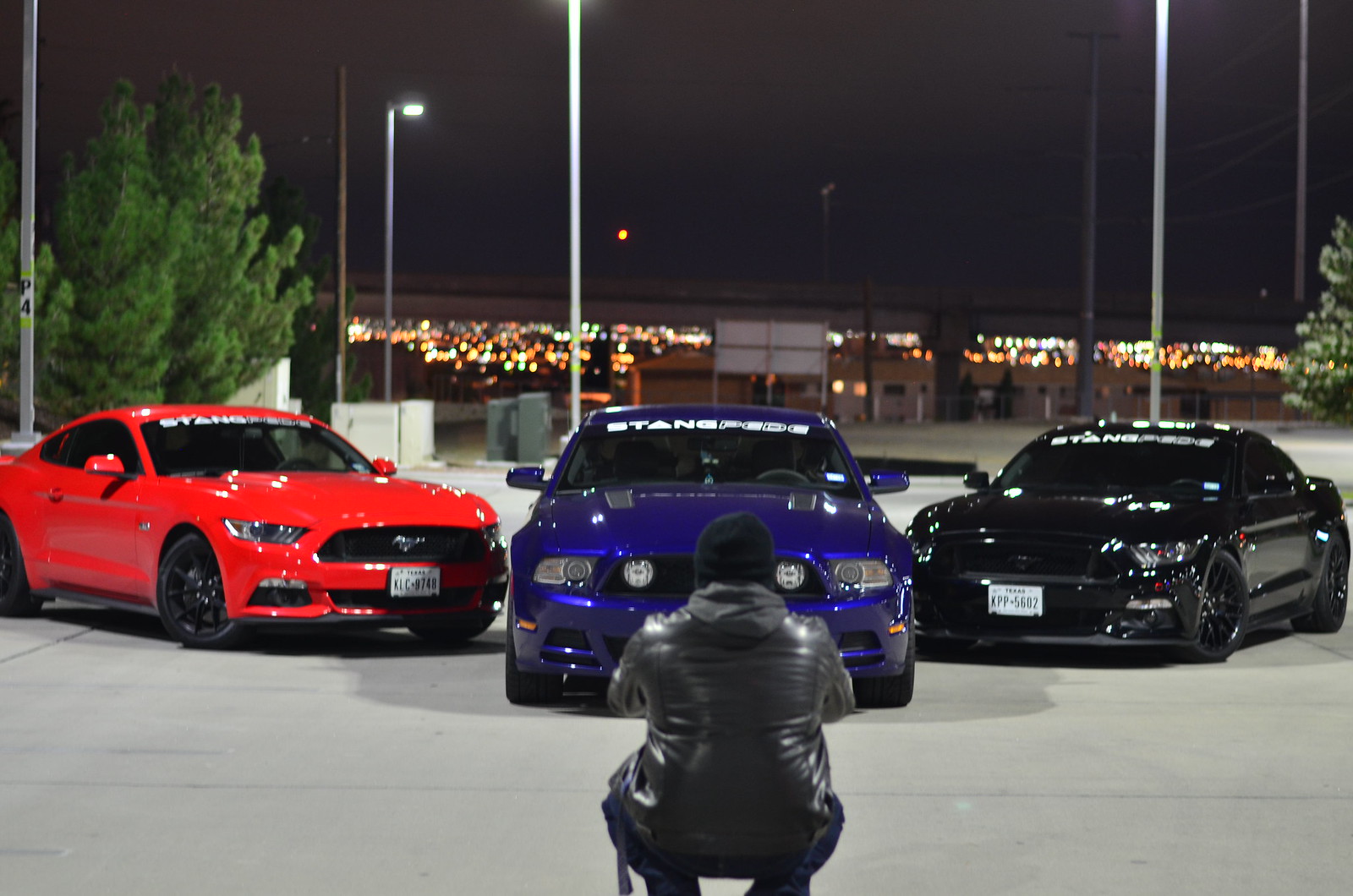In this nighttime photograph taken in a well-lit parking area, a young man is crouched down, intently focused on taking a picture of three cars arranged in a dramatic V-shape. The young man, seen from the back, is dressed in a black leather jacket, black pants, a black beanie, and a grey hoodie, with a lanyard visible from his left hip. He appears to be photographing the blue car that is parked head-on in the middle. To the left of the blue car is a striking red Mustang with white writing across the top of its windshield, while to the right is a sleek black sports car, both angled to form a V. The ground is cement-colored and dotted with light poles that cast a glow over the scene. In the background, the city lights twinkle like blurry dots against the night sky, and two pine trees are visible in the upper left corner, adding to the serene, yet urban ambiance of the image.